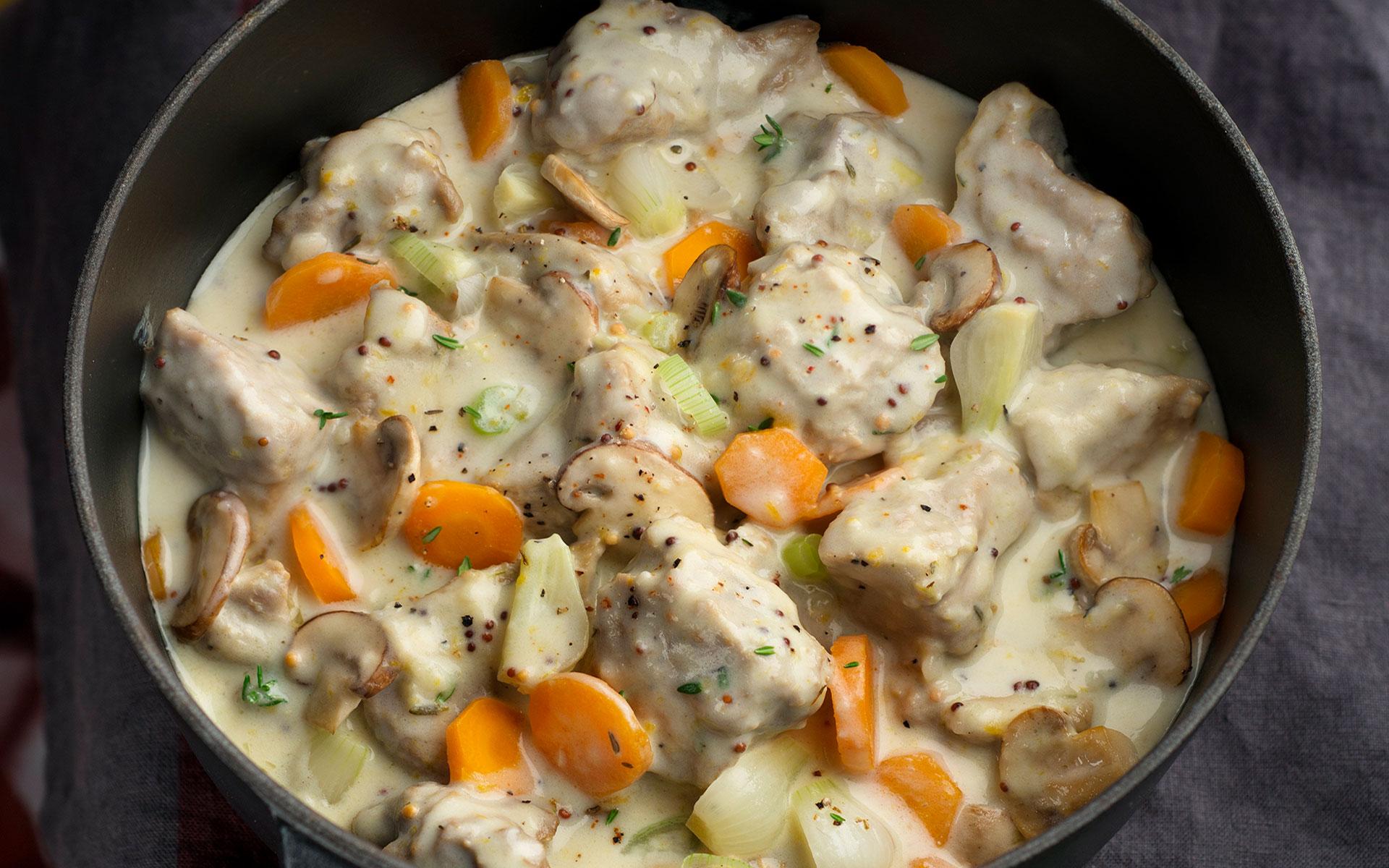This is a close-up photograph of a creamy chicken stew in a dark, almost black, cast iron pot. The pot is positioned on a grayish colored tabletop, with a dark cloth napkin on the right-hand side. The thick, white sauce with a slight yellowish tinge envelops chunks of tender chicken breast, sliced light brown mushrooms, and sliced bright orange carrots. There are also noticeable pieces of onion, cut into eighths, as well as quarters of celery and possibly chunks of garlic. The stew is seasoned with black pepper and garnished with chopped green herbs, likely parsley or chives, adding a fresh green contrast to the dish. The creamy texture of the sauce and rich combination of chicken and vegetables give it a hearty and appetizing appearance.